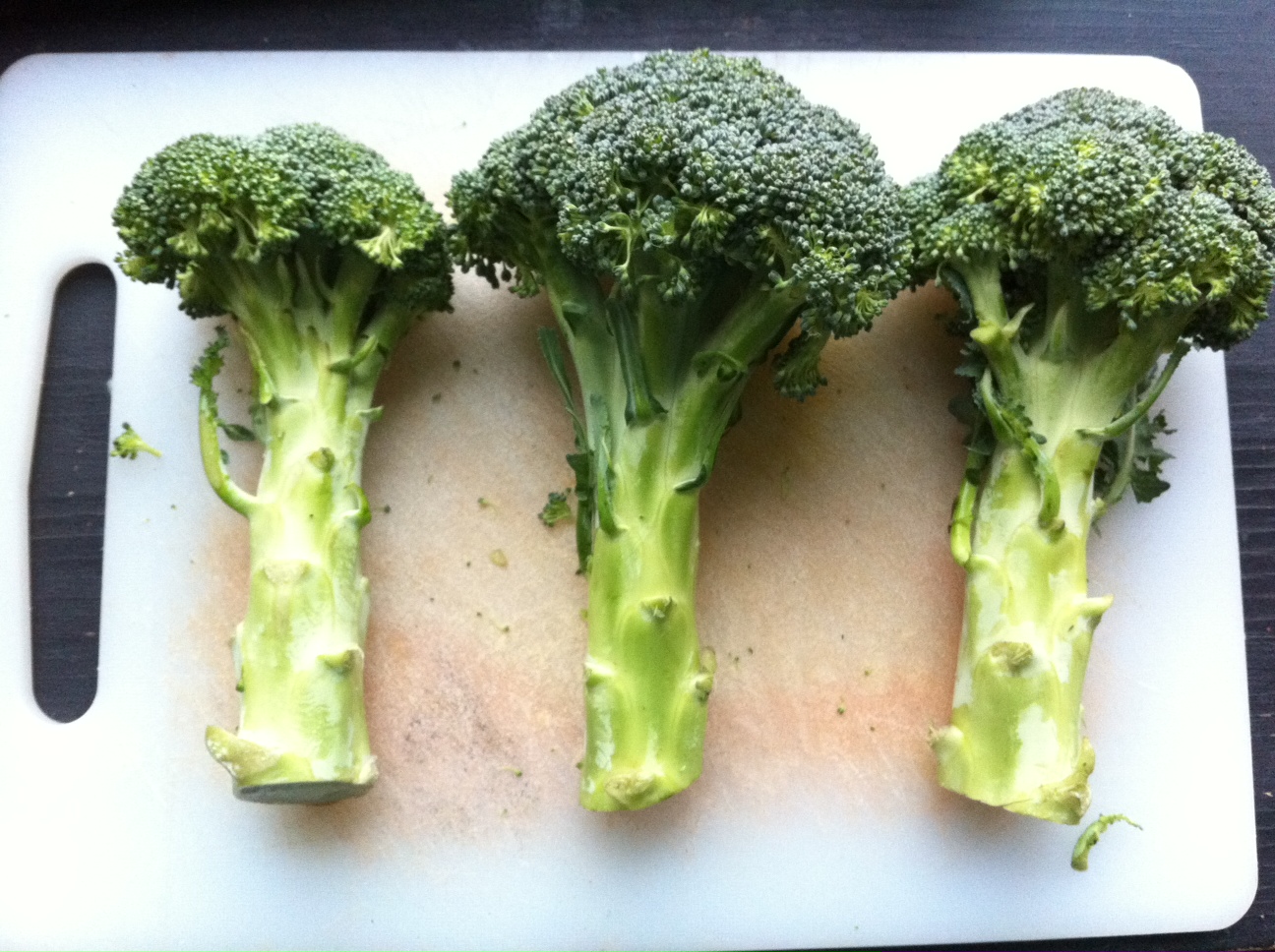A close-up, color photograph captures three stalks of broccoli of various sizes arranged horizontally on a well-used, rectangular white cutting board. The broccoli stalks display a gradient from light green at the base to dark green at the tops, which resemble the closely packed leaves of a tree. Notably, the center of the cutting board bears orange and brown stains, indicative of frequent use. The board features a small cylindrical cutout for hanging and rests on a black-stained wooden countertop, as evidenced by the visible lines denoting the wood grain in the background. This image, with its focus on the broccoli, could easily serve to showcase fresh produce recently purchased, perhaps from a supermarket or farmer's market.